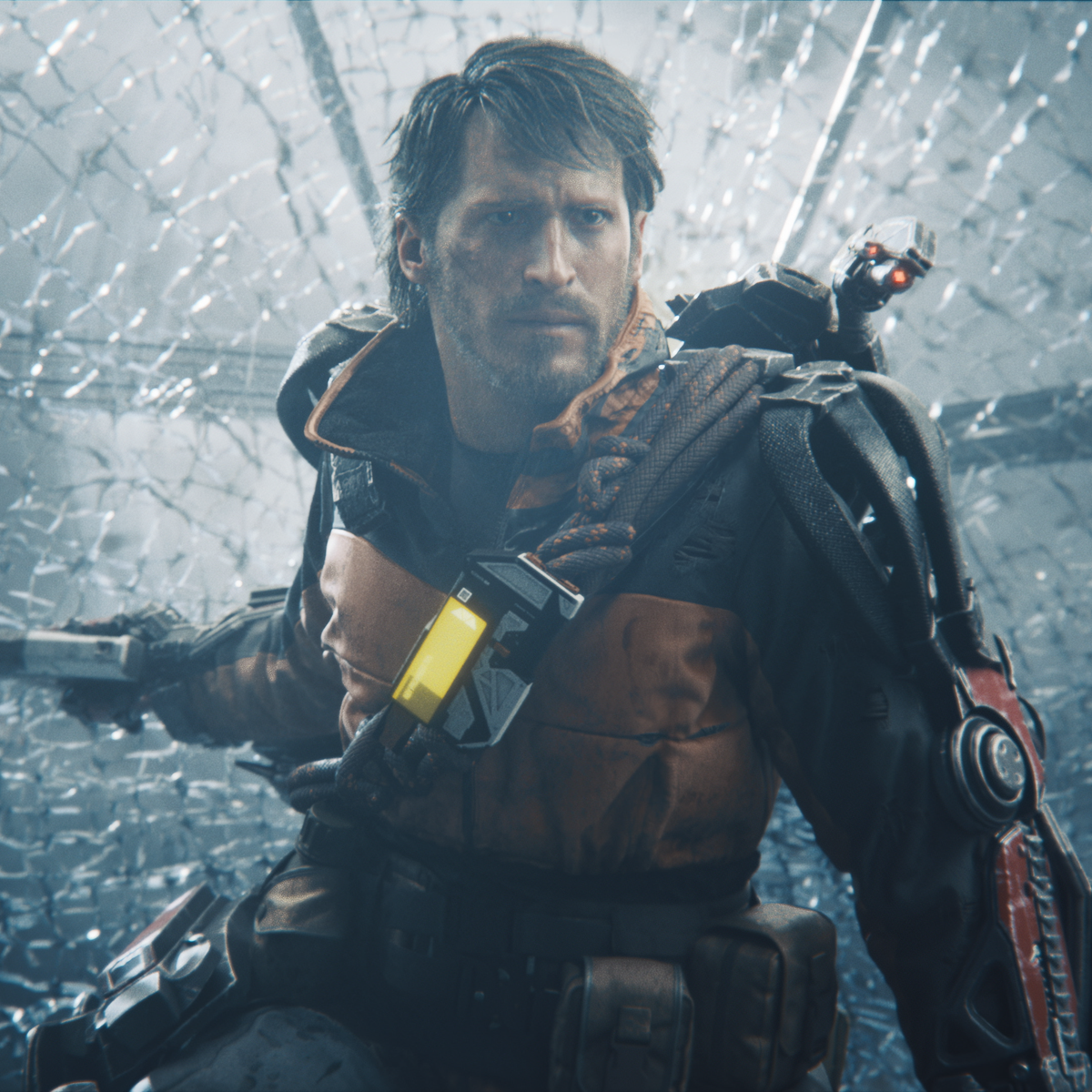This square-shaped photograph, approximately six by six inches, captures a detailed and intense scene featuring a Caucasian male character who appears to have stepped out of a movie or a video game. The man, visible from the waist up, has straight brown hair swept to the side, a stern expression under heavy brows, and sports a rough beard and mustache. He is clad in a black and orange zip-up jacket, divided with orange on the lower torso and black on the upper torso and arms. 

The character is equipped with various pieces of battle gear. His right arm is extended behind him, gripping a weapon that is pressed up against a shattered glass wall. His left arm, appearing robotic and enhanced with mechanical armor and hinges, adds to the impression of advanced combat readiness. The left shoulder is accentuated with thick bundles of rope, fastened by a black and white rectangular device featuring a yellow light.

Behind the man's left shoulder is a small, metallic device with two glowing red eyes, resembling a robot's face, suggesting an integrated artificial intelligence or advanced technology. The shattered glass wall in the background, with visible light filtering through the cracks, completes the war-ready, dystopian atmosphere of the image.